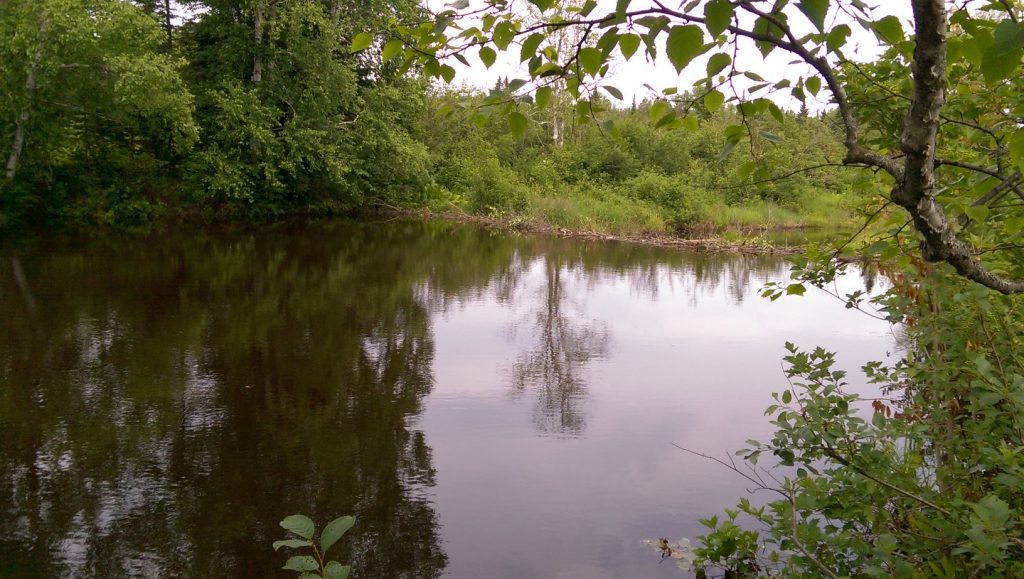This nature scene photograph captures a serene body of water, likely a lake or a pond, encircled by lush and dense greenery. To the left side of the image, vibrant emerald green bushes create a thick, dense backdrop, while the right side features an array of plants including a prominent tree, whose branches extend outward with brown and gray hues and smaller twigs. The water itself is calm, with a greenish-gray tint, and displays a captivating reflection of its surroundings, including the dense vegetation and the overcast sky. The sky, which appears light gray due to cloud coverage, frames the top of the image, with some debris or sticks visible near the water's edge. Overall, the scene is a harmonious blend of greenery and tranquil water, evoking a peaceful, natural ambiance.